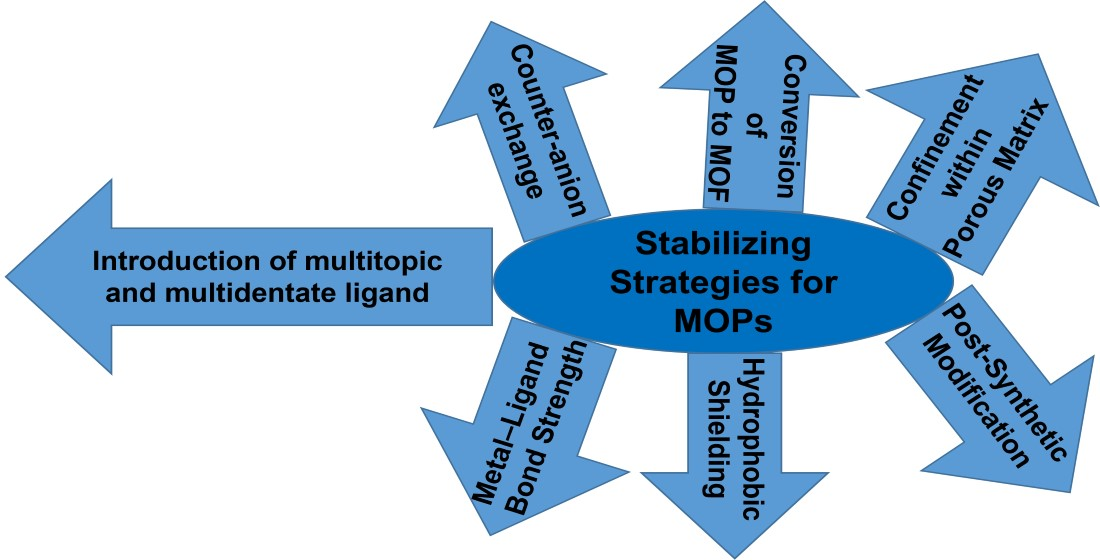The image is a detailed graphic likely used in a PowerPoint presentation, set against a white background. To the right of the center, there is a prominent blue oval with black text inside that reads "Stabilizing Strategies for MOPs." From this oval, seven light blue arrows emanate in different directions. Three arrows point upward, three point downward, and one points to the left. Each arrow has black text describing a specific strategy. The left-pointing arrow states "Introduction of Multi-topic and Multi-dentate Ligand." The three upward-pointing arrows are labeled "Counter-Anion Exchange" on the top left, "Conversion of MOP to MOF" in the center top, and "Confinement within Porous Matrix" on the top right. The downward-pointing arrows are labeled "Metal-Ligand Bond Strength" on the bottom left, "Hydrophobic Shielding" in the center bottom, and "Post-Synthetic Modification" on the bottom right. The text on the arrows is aligned with the direction of the arrows themselves, providing a structured and easily readable format.